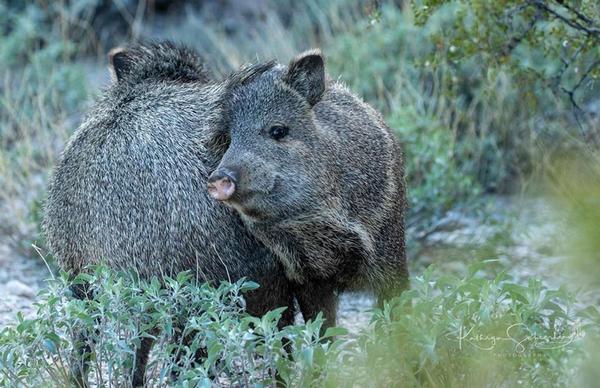In this daylight photograph of a natural scene, a unique, pig-like mammal is at the center, distinguished by its round, pink snout and dense, bristly fur, with shades of brown, gray, and tan, intermixing to give a slightly patchy appearance. The creature stands with its body pointed to the right, but it has turned its head forward, possibly rubbing its head against another similar creature beside it, giving the impression of two animals in close contact. Its face, with upright ears and small black eyes, is clearly visible. The mammal is surrounded by tall vegetation, including bushes, ferns, and grasses, which reach up past its legs. Underneath, patches of bare dirt and rocks are visible. On the top right corner of the image, a tree branch with small leaves stretches across. A white photographer's logo, in cursive script, is imprinted at the bottom right corner. The logo includes a name, but the contrast with the background makes it hard to discern, with initials likely being K and S.